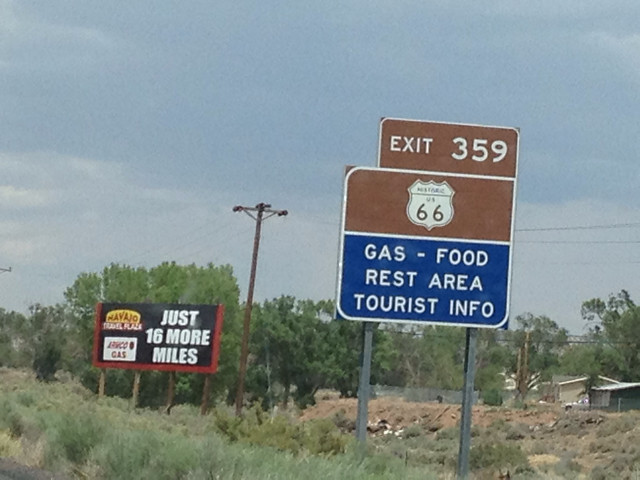This image, a color photograph with muted, almost faded hues, captures a road scene dominated by two prominent signs. In the foreground, slightly right of center, a large square sign is mounted on two grey metal poles. This sign is divided into distinct sections: the top portion is brown with a white border, featuring an emblem of US-66 and a smaller brown rectangular sign above that reads "EXIT 359" in white capital letters. The lower portion of the square sign is blue with white capital letters listing "GAS, FOOD, REST AREA, TOURIST INFO".

To the left of this sign, approximately 10 feet behind it, stands a shorter rectangular sign atop wooden posts. This black sign is outlined in red on three sides and bears white text, "JUST 16 MORE MILES," and an emblem resembling a hamburger on the left. A small white rectangle with red writing, illegible in the image, is placed at the bottom.

The backdrop is a serene landscape with a clear blue sky streaked with wispy clouds, a line of trees just below the horizon, and a utility pole with wires strung across the right side of the photograph. The foreground is a mix of green grass and barren patches of earth, with a modest one-story house visible in the bottom right corner. This combination of natural and constructed elements provides a scenic yet rustic atmosphere.